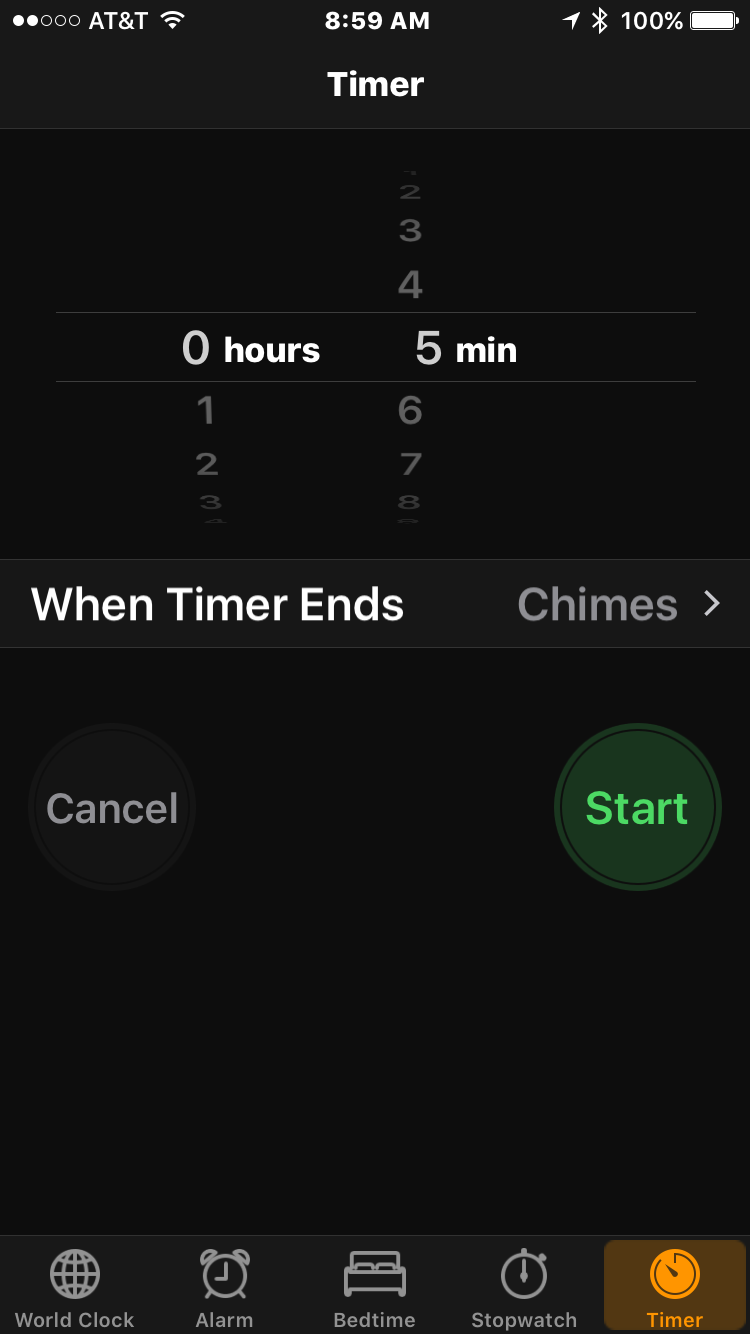**Descriptive Caption:**

The screenshot appears to be taken from an iPhone, displaying the Timer section of the Clock app. 

At the top-left corner, the signal strength is indicated by two out of five dots next to "AT&T." The current time is shown in the center as "8:59 a.m." To the right of that, icons representing airplane mode or possibly a send message function, and Bluetooth are displayed. The battery life icon on the far right shows a full charge at 100%.

Below the time, the word "Timer" is prominently displayed. Below this, two columns allow for time adjustments using the touchscreen: the left column for hours and the right column for minutes. The current setting shows "0 hours" with the numbers 1, 2, and 3 faintly visible above, and 0 minutes with numbers 1 to 8 visible below.

On the left side, a section labeled "When Timer Ends" is highlighted, which currently has "Chimes" selected as the end sound. Beneath this section, there are "Cancel" and "Start" buttons, the latter in green.

At the very bottom of the screen, there are tabs for different Clock app functions: World Clock, Alarm, Bedtime, Stopwatch, and the currently highlighted Timer tab in orange.

The screenshot effectively shows all the details necessary to set and customize a timer on the iPhone, from adjusting hours and minutes to selecting how the phone will notify you when the timer ends.